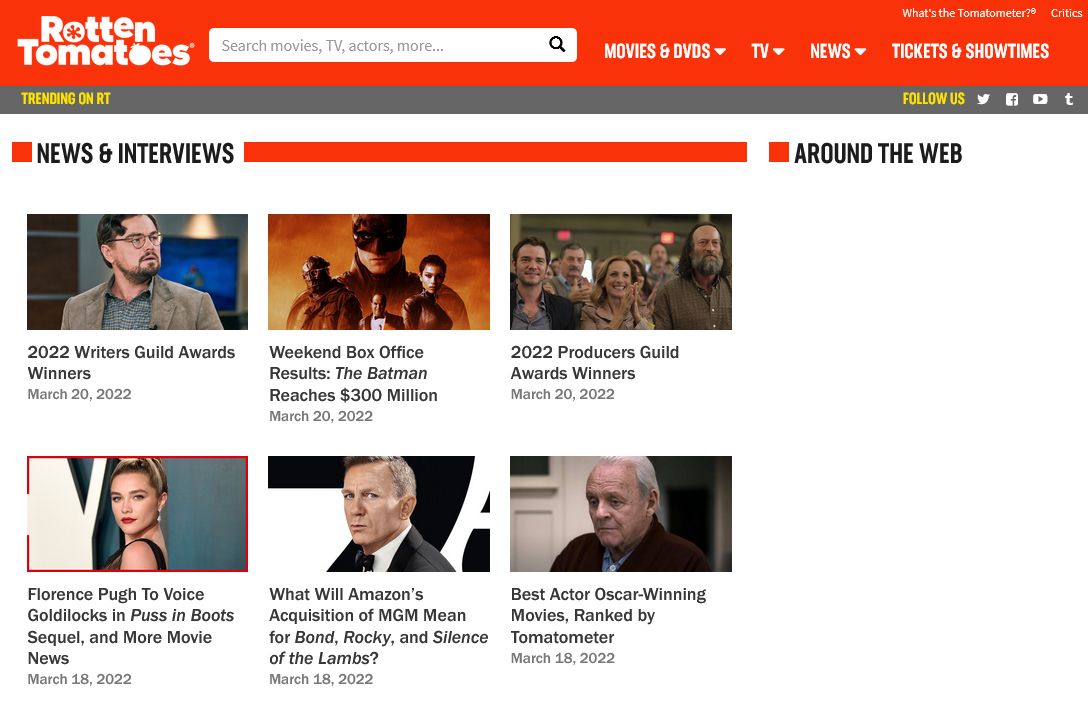This image from the popular website Rotten Tomatoes showcases a detailed layout of the homepage. At the top, a horizontal red banner features the Rotten Tomatoes logo prominently in the upper left corner. Adjacent to the logo is a white search bar, followed by navigation tabs labeled Movies, DVDs, TV, News, Tickets, and Showtimes. In the upper right corner, there is a section labeled "What's the Tomatometer?" with a question mark, and it includes a reference to Critics.

Beneath the red banner, a thin gray bar displays in yellow the text "Trending on RT," and to the right of that, also in yellow, is the phrase "Follow Us." This section includes icons for Twitter, Facebook, YouTube, and TikTok. Below this, there are sections labeled News and Interviews, as well as Around the Web, with content tiles displayed underneath.

There are six prominent tiles, each featuring different headlines:  
1. "2022 Writers Guild Awards Winner"  
2. "Weekend Box Office Results: The Batman Reaches $300 Million"  
3. "2022 Producers Guild Award Winners"  
4. "Florence Pugh to Voice Goldilocks in Puss in Boots Sequel"  
5. "What Will Amazon's Acquisition of MGM Mean for Bond, Rocky, and Silence of the Lambs?"  
6. "Best Actor Oscar-Winning Movies Ranked by Tomatometer"